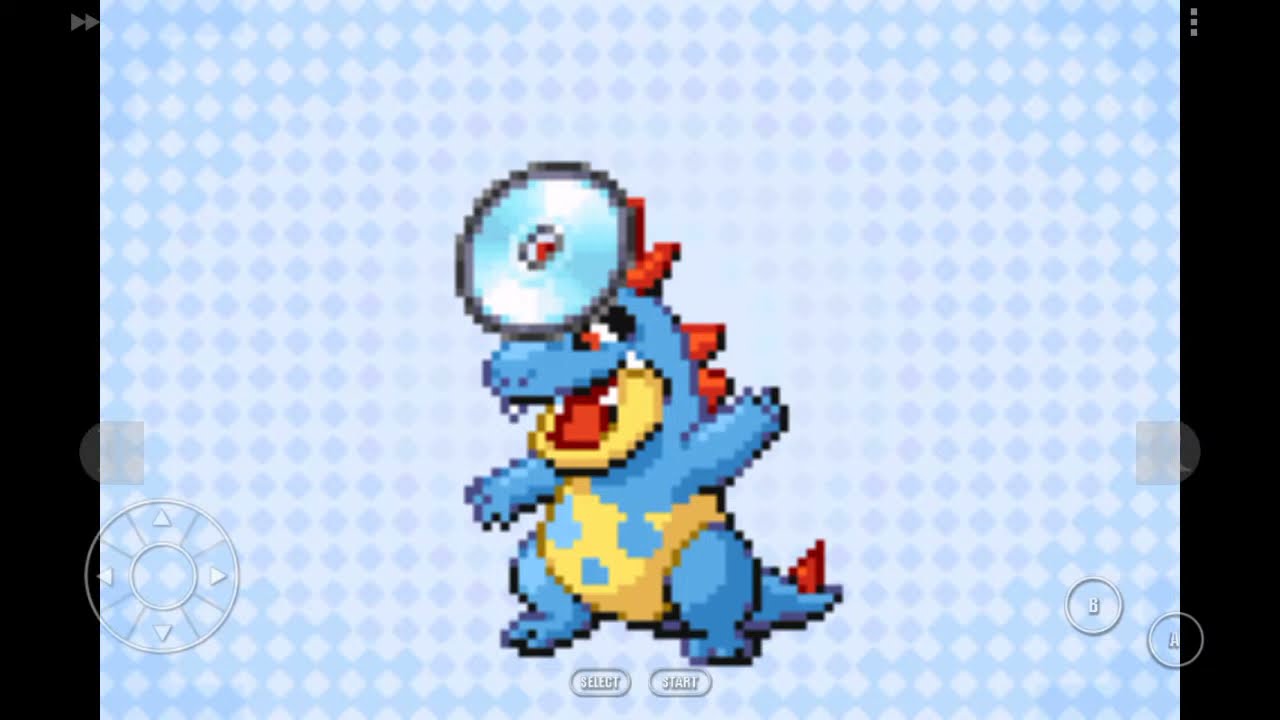The image depicts a screenshot from an old video game, featuring a pixelated, low-bit illustration of a cheerful, blue dinosaur-like cartoon character with a yellow belly adorned with blue polka dots. Resembling a stegosaurus, the creature has red spikes running along its back and tail. It stands upright on its hind legs, with one arm raised towards the top right and the other arm extended downwards to the top left. The dinosaur has an open jaw with white teeth visible from the top, a light brown chin, and red eyes gazing towards the bottom left. A notable feature on its forehead is a large silver disc, similar to the reflective mirrors occasionally worn by doctors.

The background comprises a light blue and dark blue alternating diamond grid pattern, giving a retro, 80s video game aesthetic. The bottom part of the screen includes a set of virtual control overlays, such as "SELECT" and "START" at the center-bottom, while the bottom-left corner displays a directional pad. The bottom-right corner features buttons labeled "A" and "B," with "B" positioned diagonally above "A." Additional interface elements include a fast-forward button at the top-left and three square dots at the top-right of the screen.